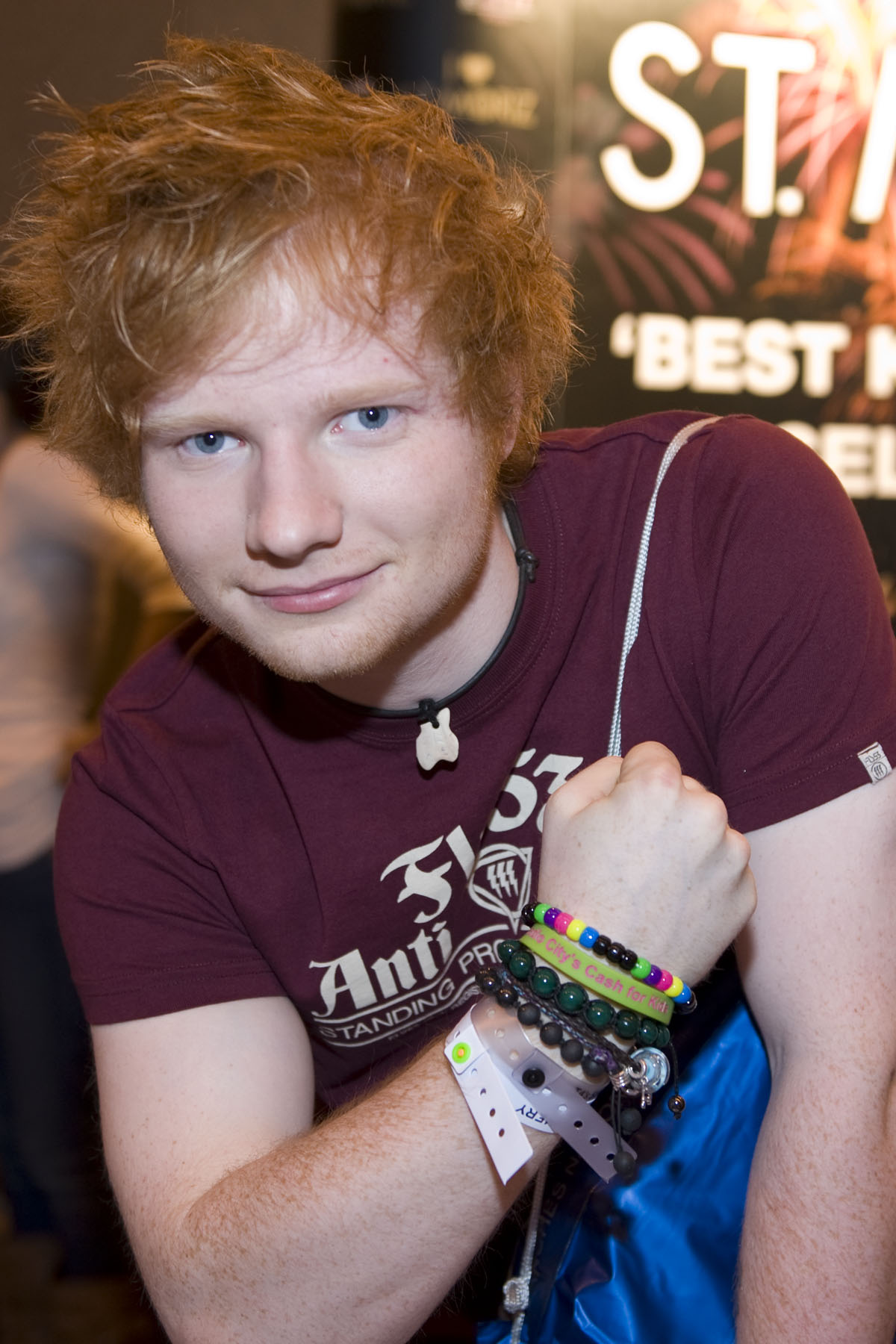The photograph is of musician Ed Sheeran. He stands at the center with his face positioned slightly to the left, the frame capturing him down to just above his waist. Sporting unkempt, tousled red-orange hair and light blue eyes, Ed has a small smile that adds a gentle expression to his face. His pale, fair skin contrasts with the dark red graphic t-shirt he’s wearing, which appears to bear multiple lines of white, cream-colored text. However, due to the angle and bends in the fabric, the words remain unreadable. Ed's right arm is outstretched in a pose as if showing off, with his hand forming a loose fist. His wrist is adorned with an eclectic mix of bracelets: a bead wristband, a yellowish-green rubber wristband, a green bead wristband, a black bead wristband, and two plastic venue wristbands. Behind him, a partially visible poster features the words "BEST" and "S&T" in white letters on a red and black background. The scene is further complemented by a vague backdrop of digital signs and an indistinct brownish background, adding depth and context to the image. Ed appears to be casually carrying something blue on his other shoulder, rounding out the relaxed and candid feel of the photograph.